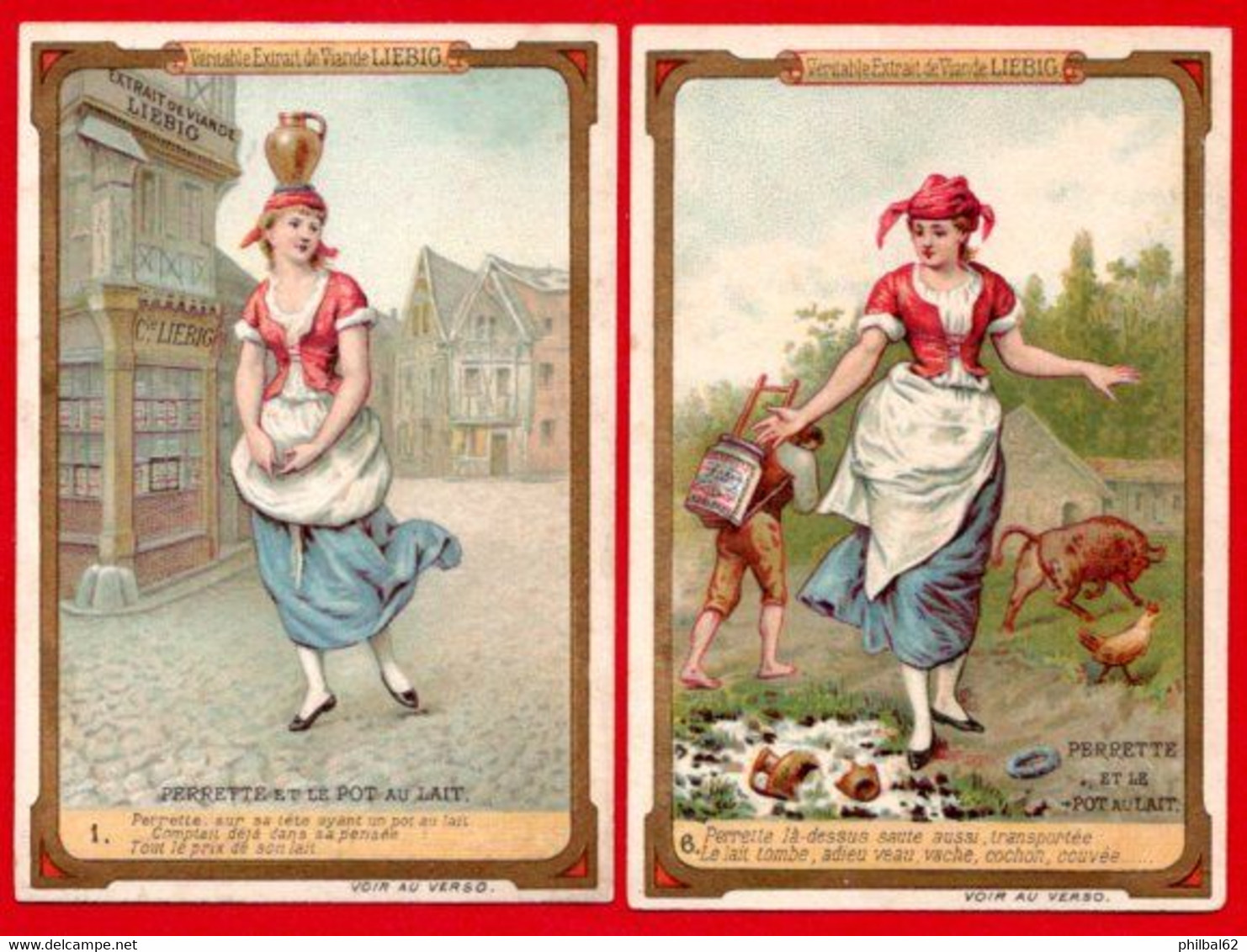This vintage image features two distinct illustrations displayed on a red background with both a white and a gold border. Each illustration portrays the same woman, showcasing a traditional scene. 

In the image on the left, the woman is dressed in a red top with fur trim that resembles a Santa Claus outfit, a white blouse, and a blue layered skirt. She wears black shoes and balances a golden jar on her head. The setting appears to be a town with cobblestone streets and buildings in the background. French text, including the phrase "Extract Day" and "Lie Big," is prominently displayed, though its exact translation is unclear. 

In the image on the right, the woman is depicted again, this time in a rural farm setting. Her red top, white blouse, and blue skirt remain the same, but the golden jar has fallen and lies broken on the ground, spilling what seems to be milk. In the background, there are various farm animals such as a pig and a chicken, and a little boy is also present. A man is seen carrying a container on his back. 

At the bottom of the images, the web address "www.dellcamp.net" is visible, suggesting the source of the printed card.